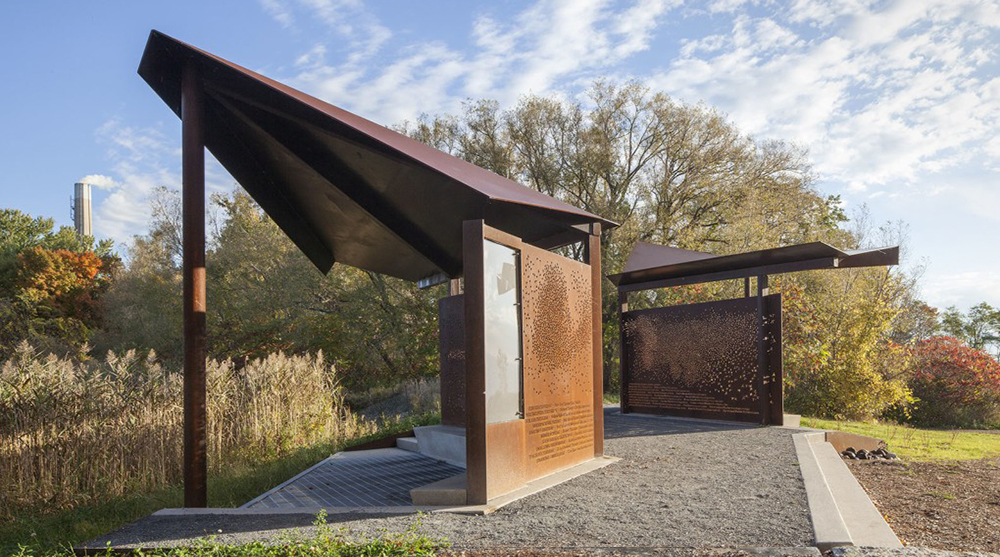This is a color photograph of an outdoor park, showcasing two striking bronze art installations situated at the center of the image. Each installation features weathered bronze panels with numerous small holes, making it difficult to discern the text and diagrams etched onto them. These panels may be commemorative or descriptive, possibly outlining historical events or local attractions. The installations are topped with artistically angled bronze roofs or canopies. Surrounding the installations, tall grass fills the left corner of the picture, and a mix of trees, some bearing orange autumn leaves, spans the background. The scene is set beneath a blue sky with scattered cirrus clouds.